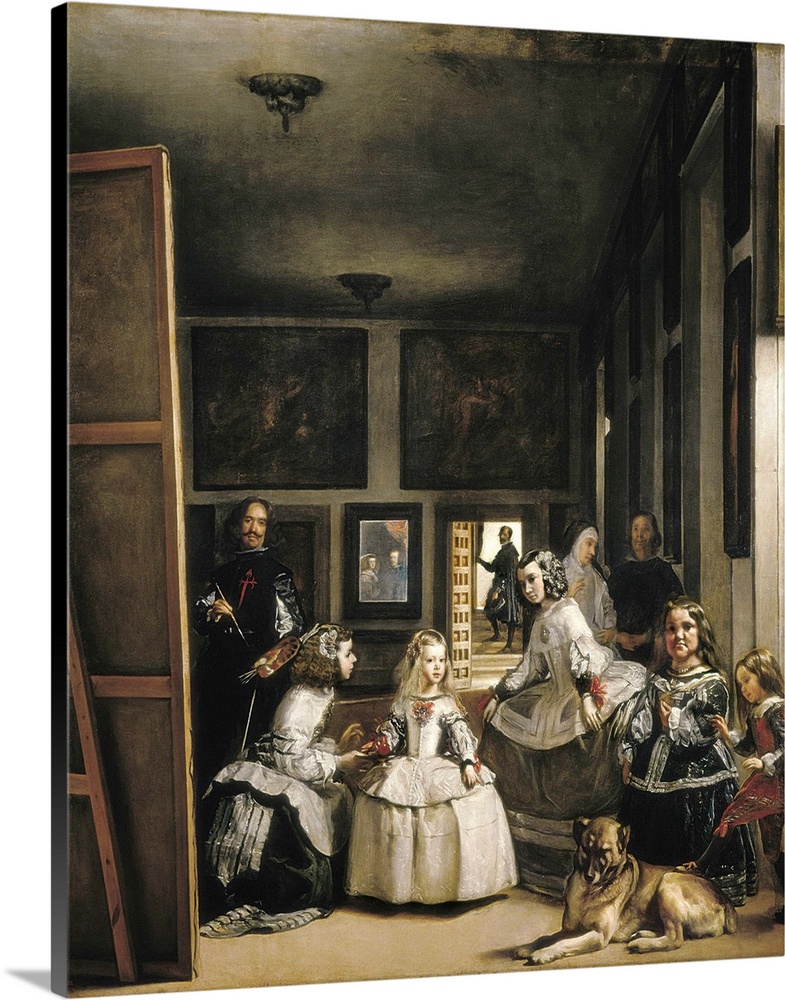The image is a detailed, old-fashioned painting or drawing characteristic of a historical or classical period, reminiscent of works like the Mona Lisa. The background of the canvas is white, and it casts a shadow, indicating it is indoors. The scene is set in a large room filled with various paintings and canvases stacked against the walls. 

In the middle foreground, there is a group of five children gathered, each with distinct features and attire; they appear to be posing for a painting. Notably, a large dog with a brown coat is laying down with its head raised and front paws extended forward. The children include a little girl with brown hair in a greenish dress, another girl with brown hair, a teenager in a white and gray dress, a blonde girl in a white dress, and another young girl talking to her, with brown hair and a white dress. 

Standing among the children is a man with a mustache and long hair, dressed in a black tunic with white sleeves and something red on the front. He appears to be an artist, possibly painting, holding something in his hand. In the dimly lit, seemingly impoverished room, one can see an open door in the background, through which another man is visible ascending the stairs. Additionally, there are more adults in the background, including a woman in a nun-like attire with a white head covering and another person in black. The left edge prominently displays the back of a large painting. The floor is a cream color, adding a subtle contrast to the dark ambiance of the room.